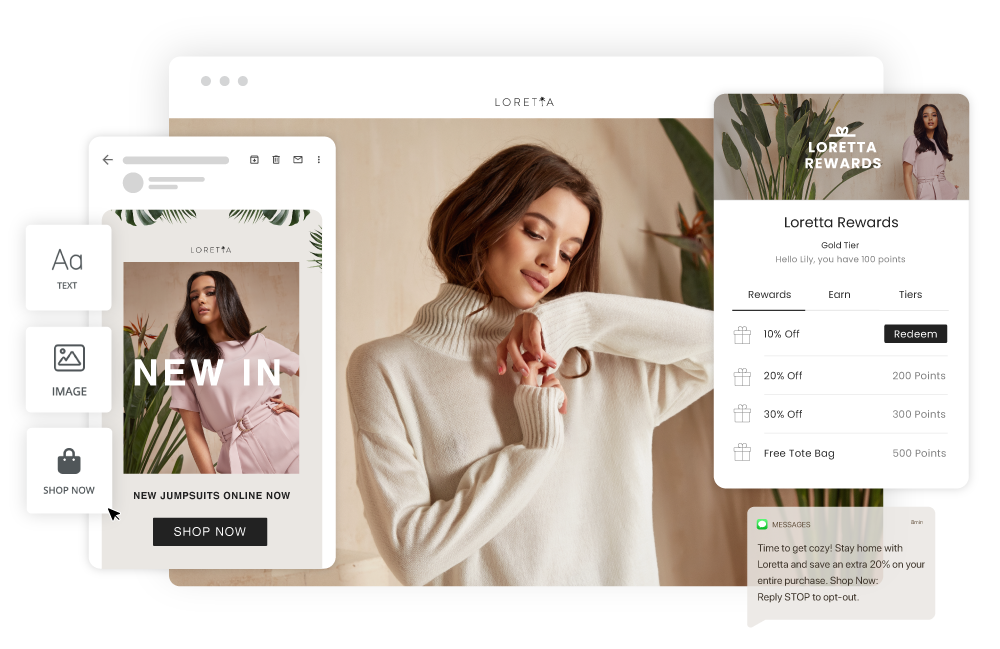The image showcases the responsive design of a web page for a brand called Loretta, illustrating how the site adapts across various devices. On the left side, there's a mobile version featuring a smaller image of a female model on the front cover, accompanied by a "Shop Now" button and some other details tailored to the phone's screen size. In the center, there's a standard desktop view with a prominent image of a woman admiring a sweater, representing the typical browsing experience on a computer. On the right side, the tablet version is displayed, slightly larger than the mobile view but smaller than the desktop, highlighting "Loretta Rewards" and some text and image elements that optimize the tablet experience. This setup demonstrates the webpage's adaptability and functionality across different devices, ensuring a seamless user experience whether accessed via phone, tablet, or desktop.